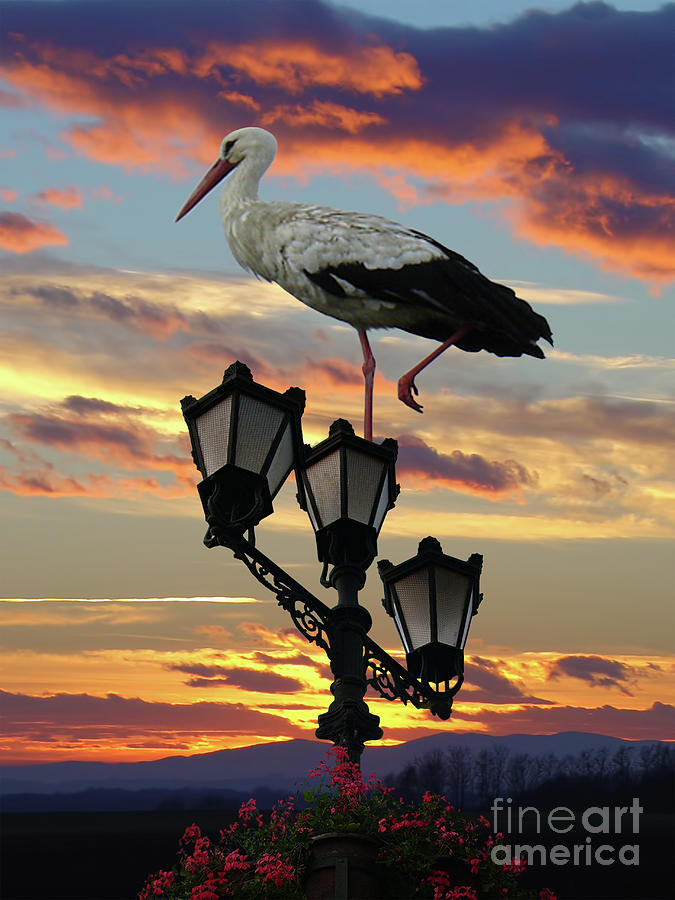This image from Fine Art America captures a tranquil moment of a large bird, possibly a heron or crane, perched on a three-light lamppost. The bird, which stands on one leg on the middle light, has distinctive white feathers covering its head and upper body, transitioning into black feathers towards the tail. Its long, pointed yellow beak faces left, adding to its statuesque appearance. The sky behind is a stunning tapestry of purple, orange, and gray hues, indicative of a dramatic setting sun. Below, the scene is framed with pink flowers, distant mountain outlines, and a hint of grass, though these elements are secondary to the primary focus on the bird and the vibrant, multi-colored sky. The bottom right corner of the image bears the Fine Art America watermark, solidifying its artistic intent.